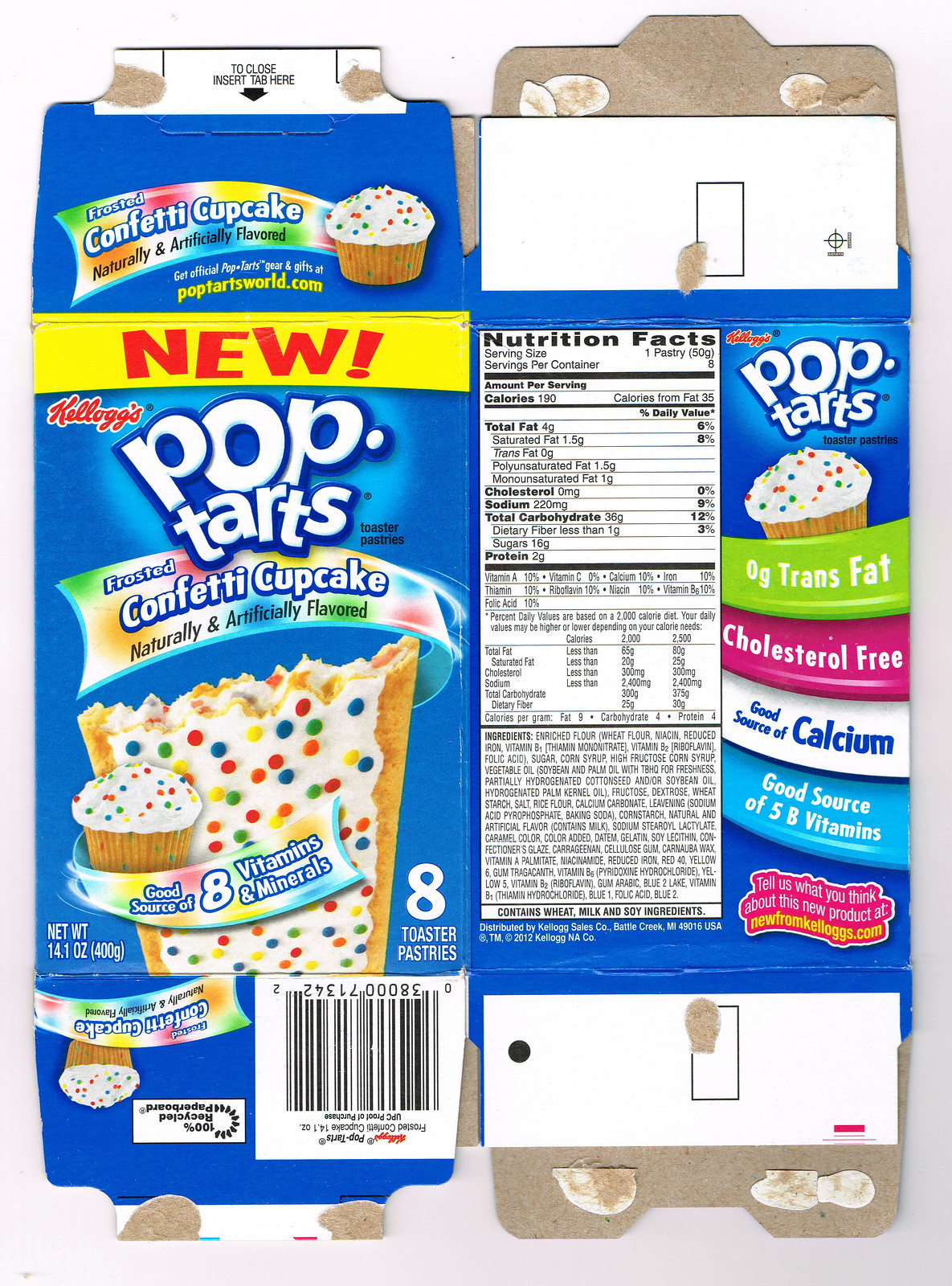This image captures a flattened Pop-Tarts box, prominently featuring the frosted confetti cupcake flavor. The front of the box, which is predominantly blue, showcases the Pop-Tarts logo in large white, cartoon-style letters. Just below, a rainbow band highlights the confetti cupcake flavor, and there's an image of a partially eaten Pop-Tart alongside a small cupcake with white frosting and colorful sprinkles.

A yellow banner at the top announces the new flavor in bold red letters with an exclamation point. The box touts its nutritional benefits, stating "8 vitamins and minerals" within a rainbow band encircling the Pop-Tart image. Near the bottom left, there's a UPC code and a note indicating the box is made from 100% recycled paperboard.

On the back of the box, which is also visible due to the flattened state, further nutritional facts are listed on the left side in various colored bands: green for zero grams trans fat, pink for cholesterol-free, white for a good source of calcium, and light blue for a good source of B vitamins. Additionally, there is a pink flag encouraging consumers to provide feedback about the new product at "newfromkelloggs.com." The entire box's design is accented with vibrant colors and additional branding details, including Kellogg’s logo in small red letters on the top right. The box appears visibly flattened, showing glue seams and creases.